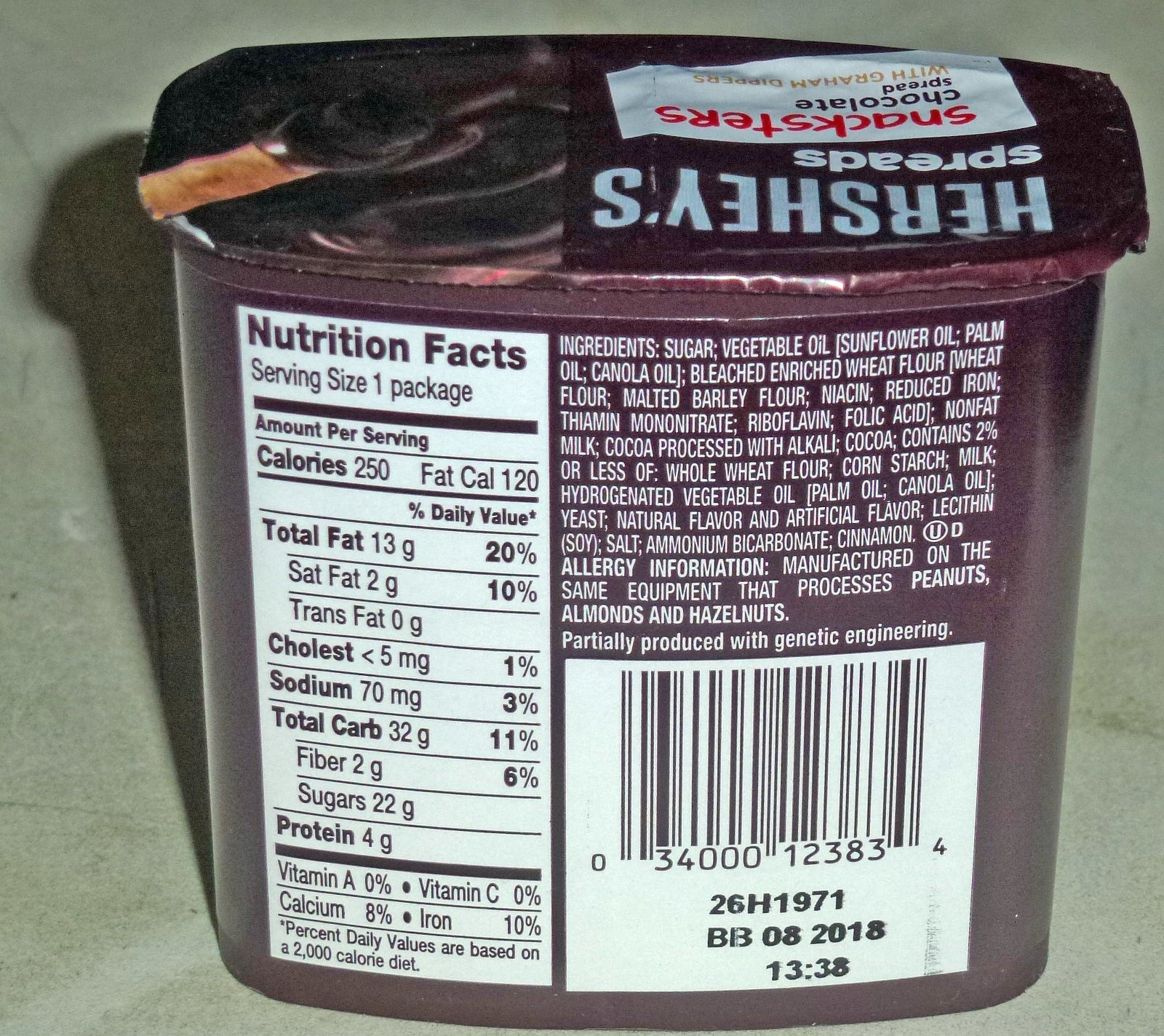This color photograph showcases the back of a Hershey's chocolate spread container, designed with a dark brown lid featuring white lettering that reads "Hershey's Spreads." Below the lid, the product name "Snacksers" is displayed upside down in black on a white rectangle, with "Chocolate Spread" inscribed in brown. The packaging also mentions in a yellowish color something along the lines of "With..." although the exact text is obscured.

The majority of the image is taken up with the nutrition facts and ingredients list, displayed on a white background with dark brown text for clarity. The label states a serving size of one package which contains 250 calories, 13 grams of fat (including 120 fat calories), 5 milligrams of cholesterol, 70 milligrams of sodium, 32 grams of carbohydrates, and 4 grams of protein. Ingredients listed include sugar, vegetable oil (sunflower, palm, and canola oils), and bleached enriched wheat flour, among others.

Adjacent to this information, there’s a UPC barcode and an identifying number "26H1971." Additionally, the packaging has a printed expiration date of August 2018 and a timestamp indicating '1338'. The product container is embellished with a detailed image featuring a swirl of chocolate spread and a lighter tan brown cookie insert.

The surface the product is resting on appears to be light gray, providing a neutral backdrop that accentuates the product’s packaging hues and information clearly.